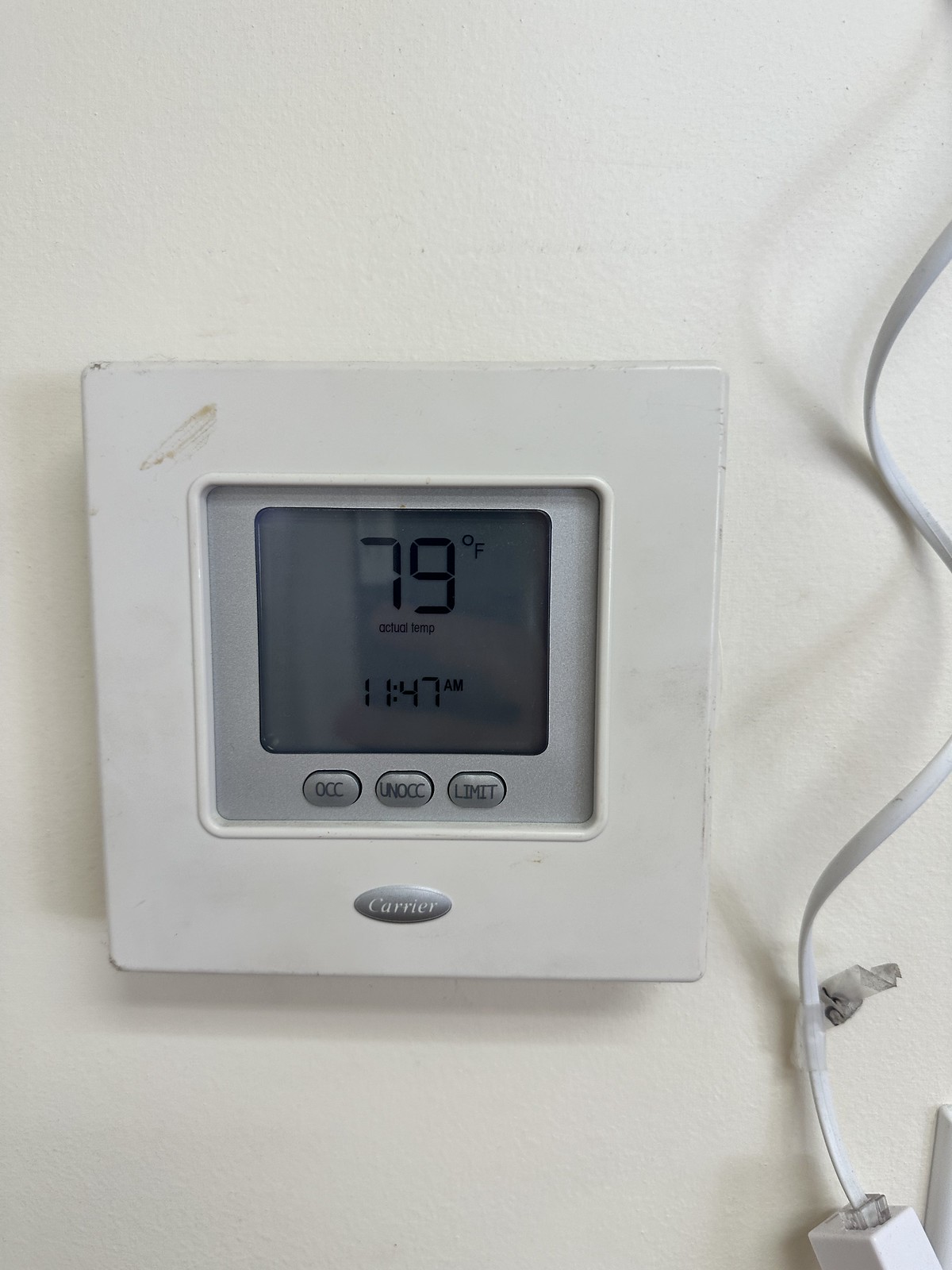This close-up photograph captures a slightly off-centered household HVAC thermostat mounted on a white wall. To the right of the thermostat, a section of a phone cord, around eight inches long, dangles down and is plugged into an adapter; the majority of the cord and adapter are out of the frame. The thermostat, displaying a reading of 79 degrees Fahrenheit, appears a bit dirty with a noticeable smudge on its top-left corner. The LCD screen in the middle of the device indicates "actual temp" beneath the temperature reading, along with the current time, 11:47 AM. Below the LCD readout are three buttons labeled "OCC," "UN OCC," and "limit." The bottom of the thermostat features the manufacturer's name, Carrier, in a small inset display within the square frame of the device.